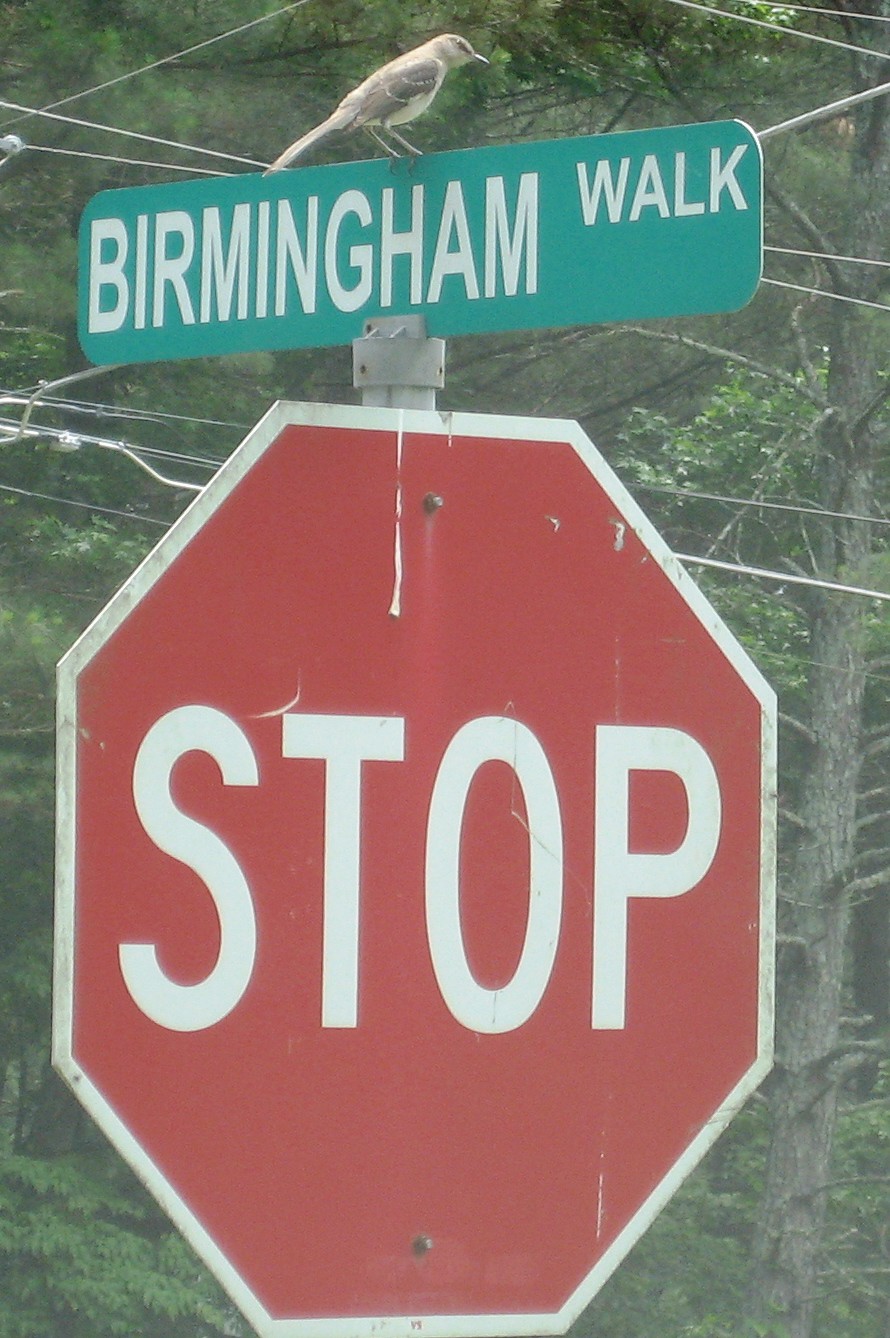This photograph captures a close-up view of a traditional octagonal stop sign with a red background and white lettering. The stop sign fills approximately three-quarters of the lower portion of the vertically-oriented image, with only the sign visible and the pole cut from the frame. Atop the stop sign is a green rectangular street sign that reads "Birmingham Walk" in white letters. Perched over the 'H' in 'Birmingham' is a medium-sized bird with brown and white plumage, likely a mockingbird, facing right. A notable detail includes a small white substance on the upper part of the stop sign, possibly from the bird. The background features a mix of trees with lush green leaves, power lines, and telephone wires.